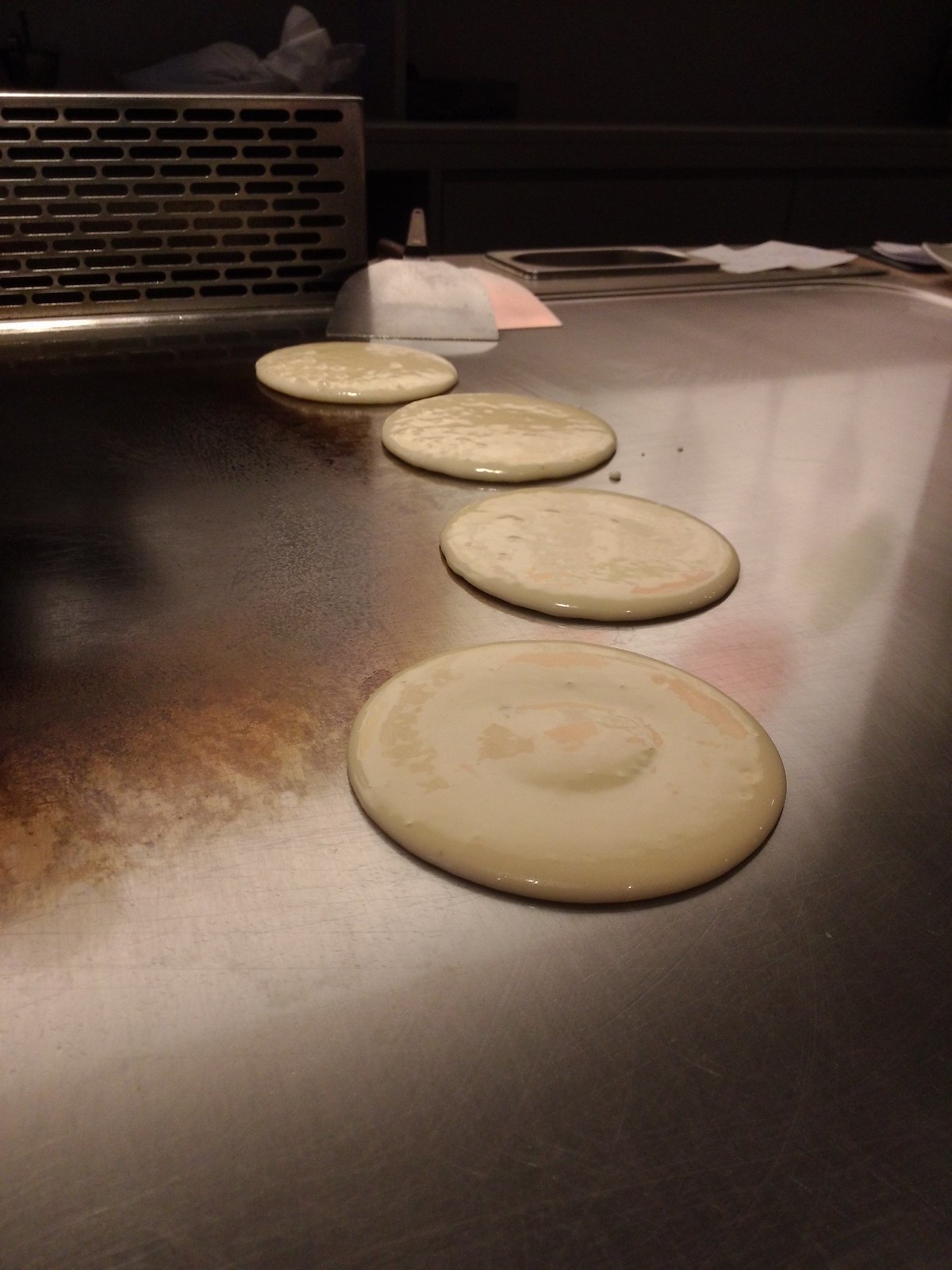The image shows a close-up of a professional, polished griddle surface, likely in an industrial kitchen or diner, with a light coating of oil that gives it a shiny appearance. On this clean, stainless-steel griddle, there are four circular pools of pancake batter lined up from the forefront to the upper left. The batter has recently been poured, suggesting the pancakes are still cooking on the bottom with their tops remaining raw. Positioned in the upper left corner of the image is a metallic air intake vent, part of the griddle's ventilation system to manage smoke and steam. To the right, next to the griddle, there are spatulas and some paper, indicating the tools the chef might use. The image primarily focuses on the griddle and uncooked pancakes, with the corners of the photo fading into a dark background, ensuring the cooking scene is the central point of interest.